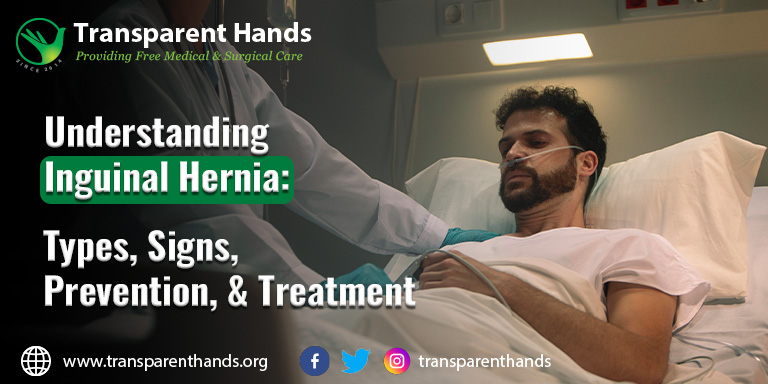The image depicts a detailed hospital scene centered around a man receiving medical care. The man, lying slightly upright in a hospital bed, has dark hair, a thick beard, and a mustache. He wears a white shirt and rests his head on a white pillow, with a nasal tube providing oxygen. His left hand rests on his midsection, while his right hand is monitored by a healthcare professional – either a doctor or a nurse – dressed in a white full-sleeved uniform, gloves, and a mask. The healthcare professional's hand is placed gently on the patient's right shoulder and midsection. 

Overlaying this scene, on the left side of the image, is extensive text and branding. At the top, a logo featuring a bird and the phrase "Transparent Hands" is displayed in white. Directly beneath, in light green writing, it reads "providing free medical and surgical care." Further down, the text discusses "understanding inguinal hernia" with "types, signs, prevention, and treatment" laid out in a structured format using white text and green backgrounds for emphasis. At the bottom, "www.transparenthands.org" appears alongside social media icons for Facebook, Twitter, and Instagram, with the handle "Transparent Hands" also mentioned. This image, possibly part of a promotional poster or ad, focuses both on the patient’s care and the medical organization's mission and services.